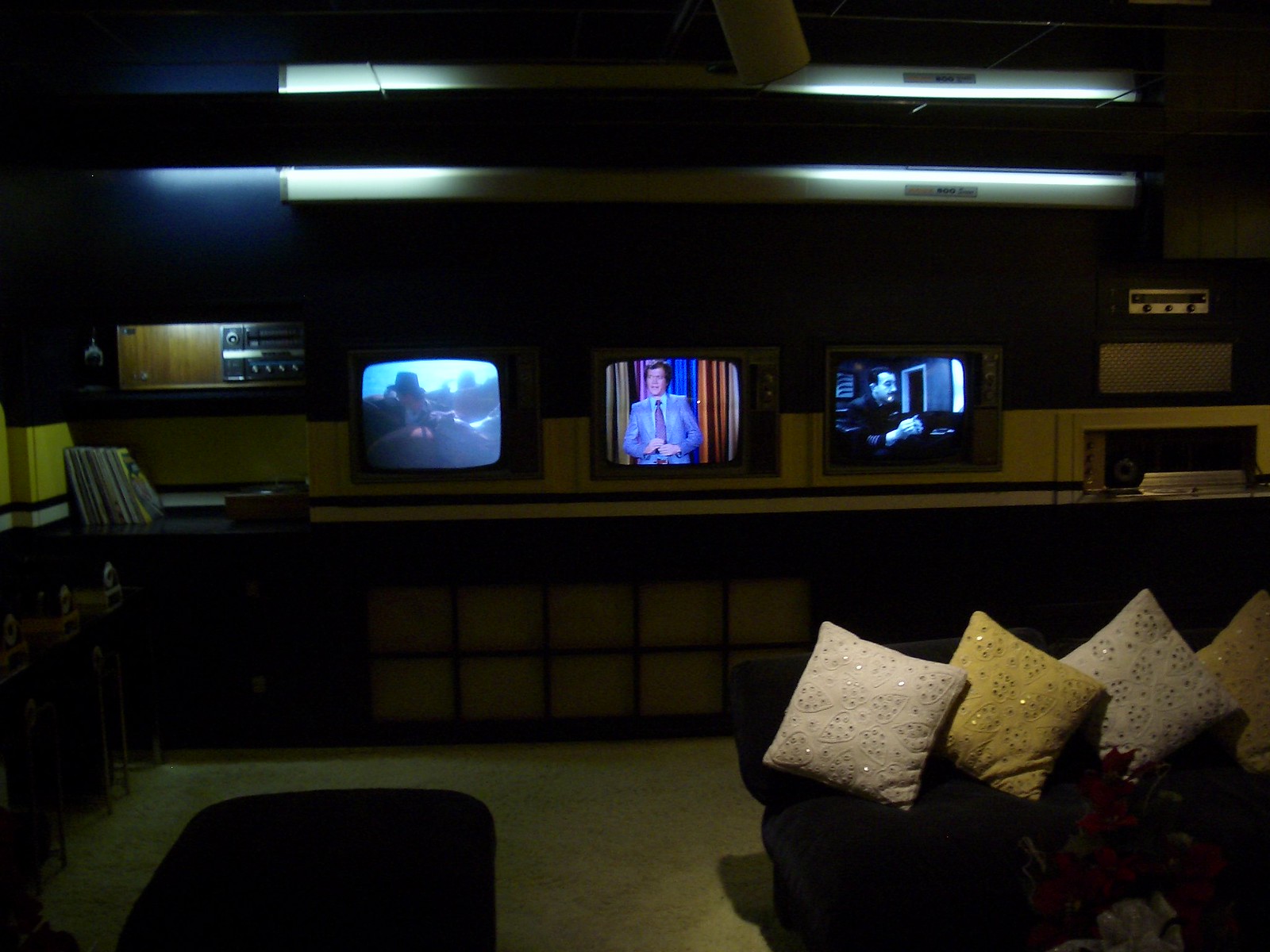The dimly lit den boasts a unique green and brown color scheme on the walls and trim, creating a cozy atmosphere. Front and center, three boxy, vintage TV sets are lined up symmetrically atop a large TV stand. Each screen displays a different image: the middle TV features what looks like an old talk show, possibly Johnny Carson, while the other two TV screens show stills from what appear to be action movies. Overhead, a pair of lights shine down on the TVs, highlighting their retro charm.

To the side, a blue couch adorned with four pillows – three beige and one yellow – offers a comfortable seating option. Adjacent to the couch, a brown old radio is built into the wall, featuring a prominent speaker at its base. A little stereo system and various electronics are placed on a desk, which is topped with some books and framed by a golden-colored floor.

In addition, a table and an ottoman occupy the center of the room. The stand that holds the TVs also features a distinctive design of a large rectangle with slats creating ten smaller squares – five on the top and five on the bottom – for added visual interest. The overall decor includes various devices and objects, seamlessly blending nostalgia with functionality.